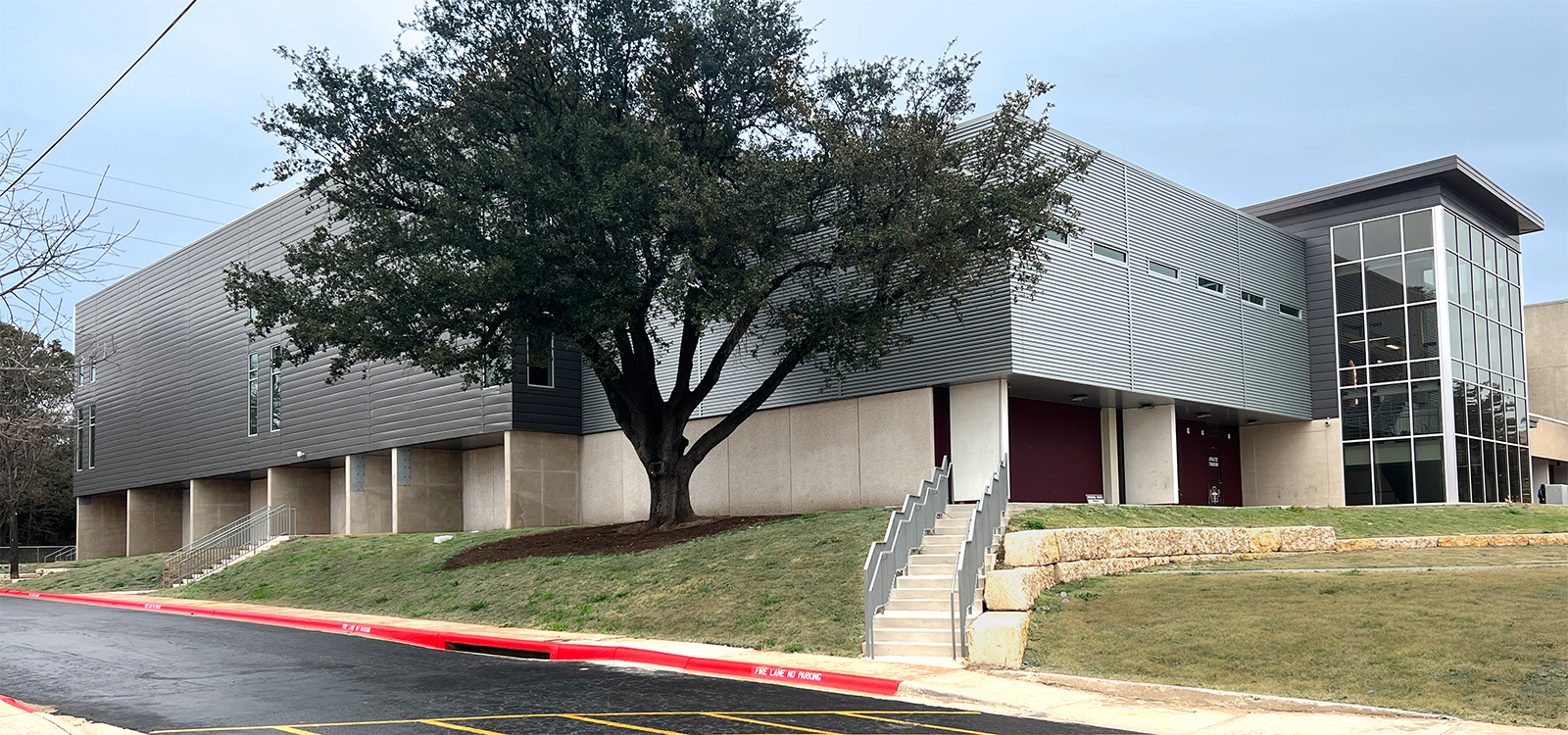This image showcases a recently constructed or remodeled modern building with a distinct, contemporary design. The structure is primarily composed of gray concrete and features sleek metal siding. It has a squared or rectangular shape with a completely flat roof. The facade includes an expansive, towering glass front, indicating it might be a business center rather than a residential building. 

The building is elevated slightly on a green grassy hill and is accessible via concrete stairways with silver railings. The prominent exterior windows include both horizontal and vertical narrow designs, adding to its modern aesthetic. 

In front of the building, there is a damp blacktop driveway or parking area, indicative of recent rain, accompanied by a yellow crosswalk. A red-striped sidewalk surrounds the building, clearly marked with a "No Parking" message. A large tree, fully leaved with a dark brown trunk, stands prominently in the foreground, adding a touch of nature to the otherwise sleek, industrial setting. Overall, the scene is outdoors, under a very cloudy sky.